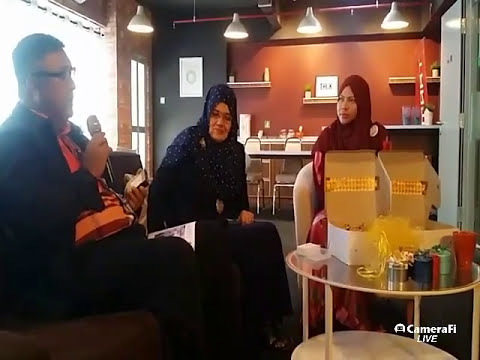The image from Camera 5 Live captures a detailed scene inside a restaurant. A man, who appears to be conducting an interview for a news show, is situated in the center, holding a microphone near his mouth and a cell phone in his other hand. He is wearing black framed glasses, a dark jacket, an orange-red scarf, and black pants, with a book or newspaper resting on his knee. He is seated on a brown booth couch beside two women, both of whom have their heads covered. The woman to his right is older, wearing glasses, a dark dress, and a scarf covering her head. The woman next to her wears a red headscarf and matching red dress. They are all gathered around a small, round glass-top table filled with various items, including two open white boxes and several small containers in silver, blue, and green. The background features shelves with small plants, a painting, a window, a door, and track lighting above. The setting presents a cozy and intimate interview environment, showcasing possibly local treats or products from the restaurant.